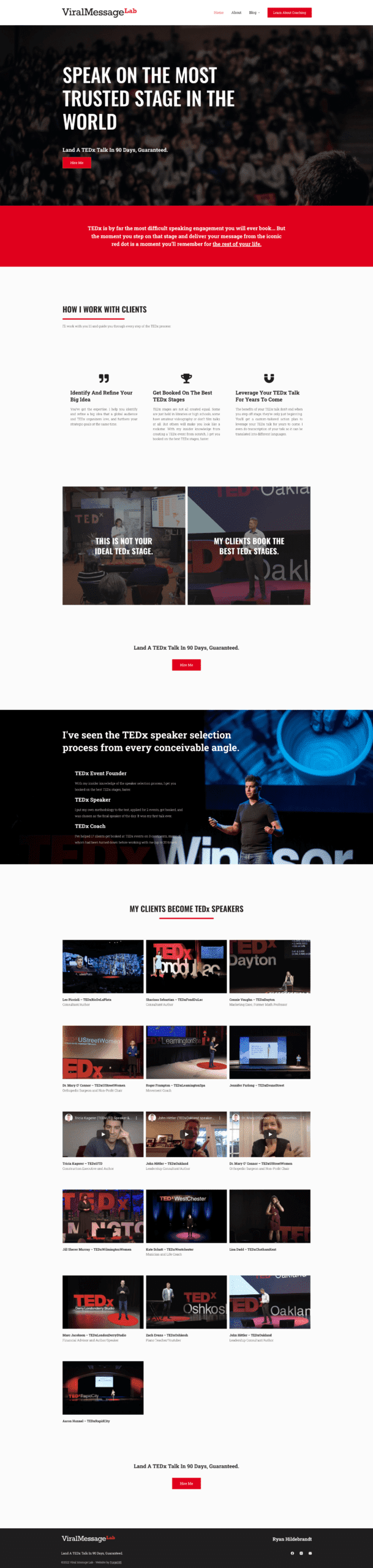This is a detailed description of a web page screenshot. 

At the top of the page, there is a white header with dark grey text on the left that reads "ViralMessageLab." The word "Lab" is slightly raised, smaller in size, and colored red. To the right, after some negative space, there is a series of navigation options: "Home" in red text, "About" in dark grey text, "Blog" in dark grey text with a dark grey triangle pointing down, and a red rectangle with white text that is too blurry to read.

Beneath the header, there is a photograph of a crowd sitting in an auditorium, with the back of a man's head visible in the bottom right corner. The photograph is darkened, creating a contrast with the large white text in the center-left that reads: "SPEAK ON THE MOST TRUSTED STAGE IN THE WORLD." Below this, in smaller white text, it says: "Land a TEDx talk in 90 days guaranteed." 

Underneath this, there is a red button with white text that is too blurry to read. Following this section, the background color changes to red, and in the center, a white paragraph of text reads: "TEDx is by far the most difficult speaking engagement you will ever book... But the moment you step on that stage, and deliver your message from the iconic red dot, is a moment you'll remember for the rest of your life." The phrase "the rest of your life" is underlined.

Further down, the background changes to white, and in the top left corner, there is black text in all caps that says: "HOW I WORK WITH CLIENTS."